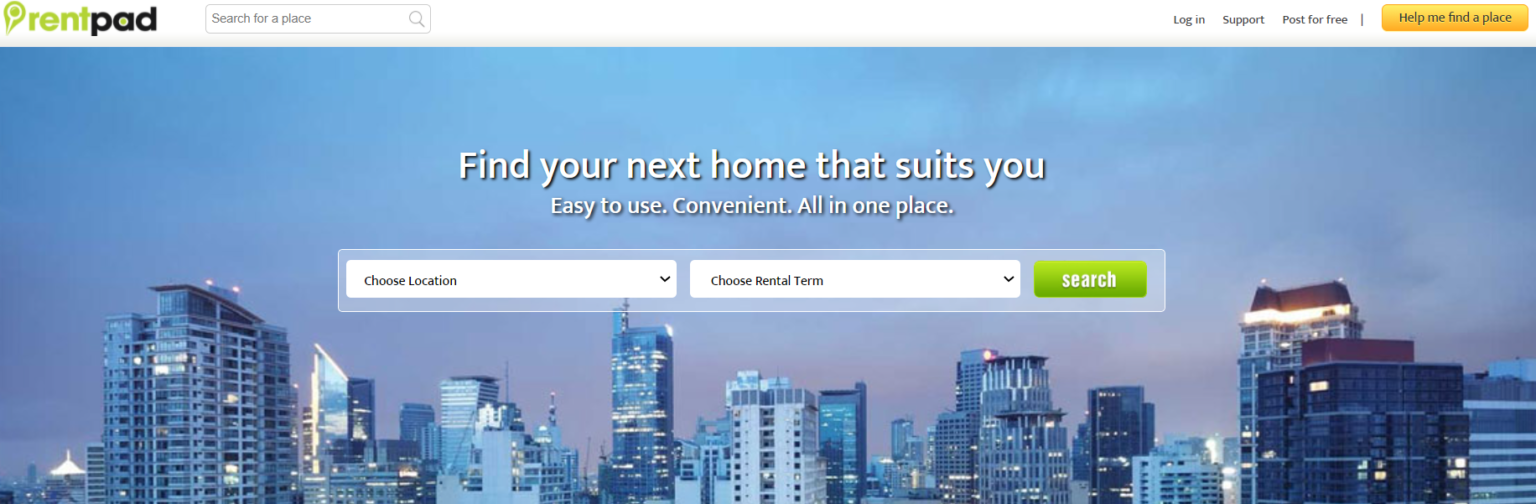In the landscape-oriented screenshot of a laptop screen, the website "Rent Pad" is prominently displayed. The upper-left corner features a green location icon followed by the "Rent Pad" logo, with "Rent" in green and "Pad" in black. Directly below the logo, there's a search bar labeled "Search for a place."

On the upper-right side, user options are listed: "Login," "Support," and "Post for free," with an orange button labeled "Help me find a place" for additional assistance.

Spanning across the next row is a large, captivating image of a cityscape at nighttime, with a light to dark blue gradient sky. The city’s skyscrapers are illuminated, though the specific city is not immediately recognizable.

Dominating the center of the screen, a header in bold font reads, "Find your next home that suits you," followed by a subheading, "Easy to use, convenient, all in one place."

Below this text, there's a large, rounded rectangle with a gray background containing interactive search options. The first button, "Choose location," is white with a black arrow. Adjacent to it, the button "Choose rental term" is similarly styled. A green button, positioned to the right, displays the word "Search" in white font.

This entire interface collectively illustrates the "Rent Pad" website, designed for easy and convenient property searching.